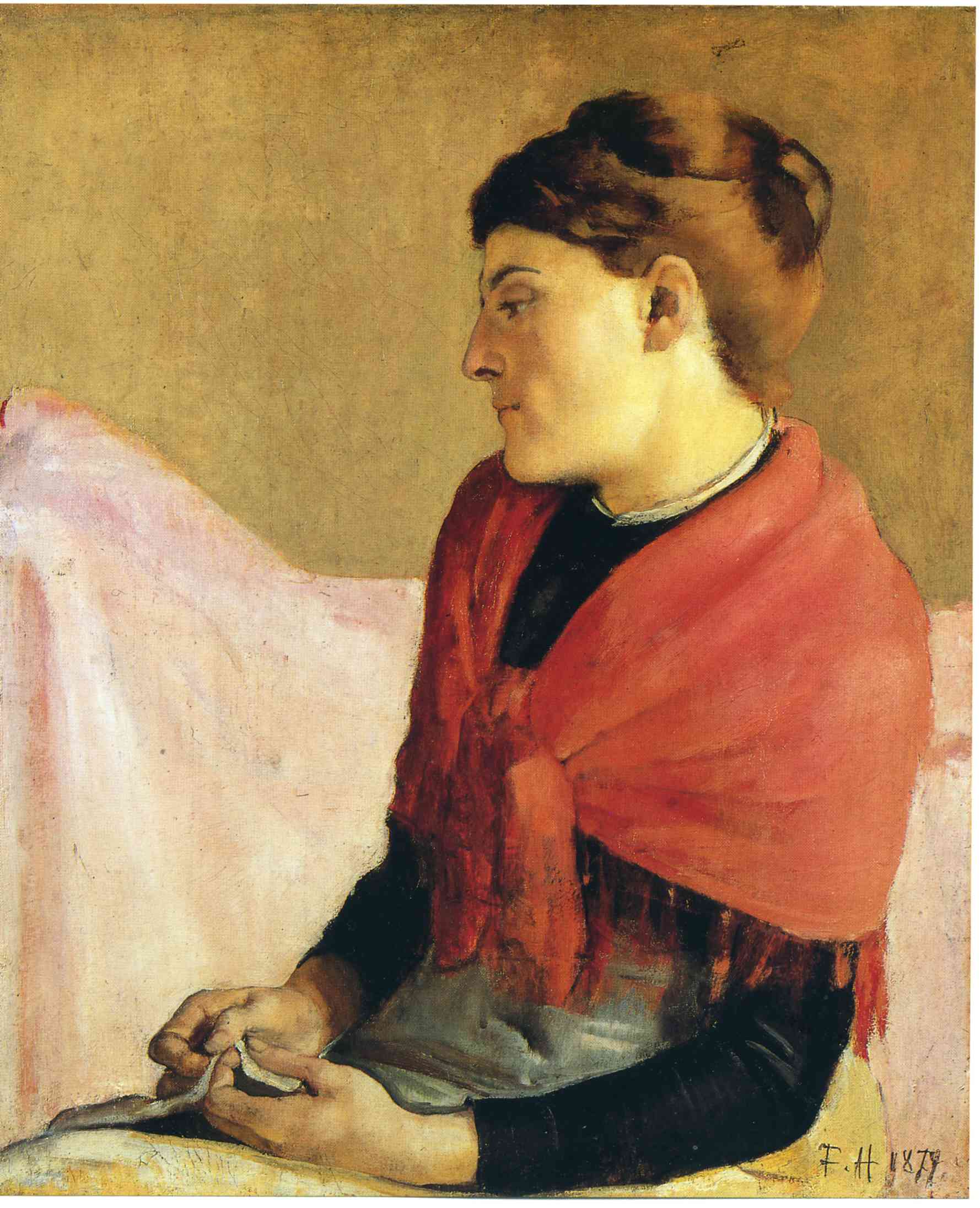The painting portrays a woman with brown, auburn hair neatly secured in a top bun, offering a side profile as she sits facing the left. She appears deep in contemplation, softly clutching a white handkerchief in her lap. A muted red, almost strawberry-colored shawl drapes elegantly around her shoulders, tied neatly at the front. Under the shawl, she wears a black long-sleeved top paired with a dress that carries a worn, yellowish hue, possibly aged. The backdrop reveals a warm tan and brown color, with a contrasting pink or white cloth draped over what could be a couch, hinting at a domestic setting. The painting is meticulously detailed, showing the wall's orangey-yellow tones and ensuring the signature "FH 1879" stands visible in the bottom right corner.